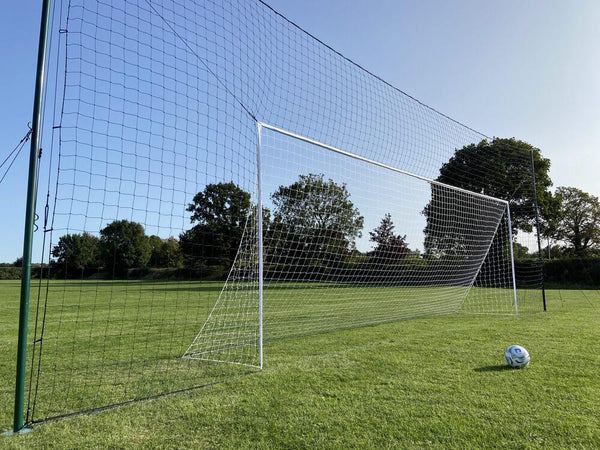The image captures a well-maintained, green soccer field with a prominent white goal post equipped with a black net. The frame of the goal post, made of metal, stands out distinctly against the field. The goal's structure is complemented by an orange frame providing additional support. In front of the goal, slightly to the right, lies a white and blue soccer ball, casting a shadow to the left, suggesting a light source from the upper right. The field's grass exhibits variations in green hues, attesting to its regular upkeep. In the background, a row of trees and shrubs define the boundary, with a clear, blue sky overhead indicating a bright, sunny day, further enhancing the sportive atmosphere of the scene.